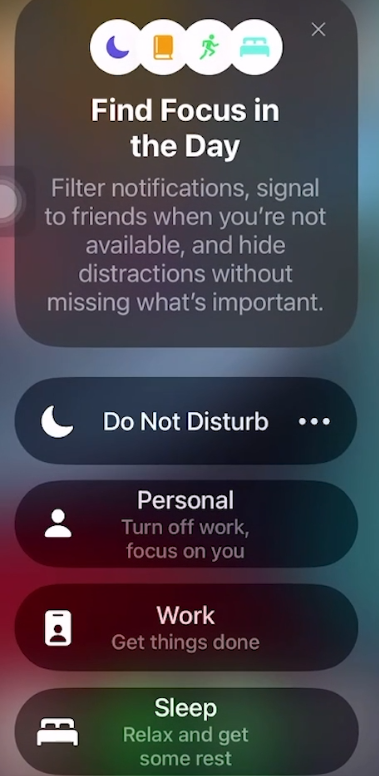The screenshot is set against a multicolored background of dark greys, reds, and gold. In the upper half of the image, there is a prominent black box showcasing several white icons, which include a moon, a book, a running person, and what appears to be a car. Below these icons is an informative text in white font: "Find focus in the day, filter notifications, signal to friends when you're not available, and hide distractions without missing what's important."

Directly underneath this text is another section featuring a moon icon accompanied by the words "Do Not Disturb" followed by three dots. This is followed by smaller boxes with specific focus modes. The first box is labeled "Personal" in white text inside a black background, with the subtitle "Turn off work, focus on you." Below that is another black box labeled "Work" with the subtitle "Get things done." The final section of the screenshot depicts a white bed icon next to the word "Sleep," with the subtitle "Relax, and get some rest."

This detailed layout effectively communicates the functions and benefits of the focus modes available, highlighting essential features to aid productivity and relaxation.